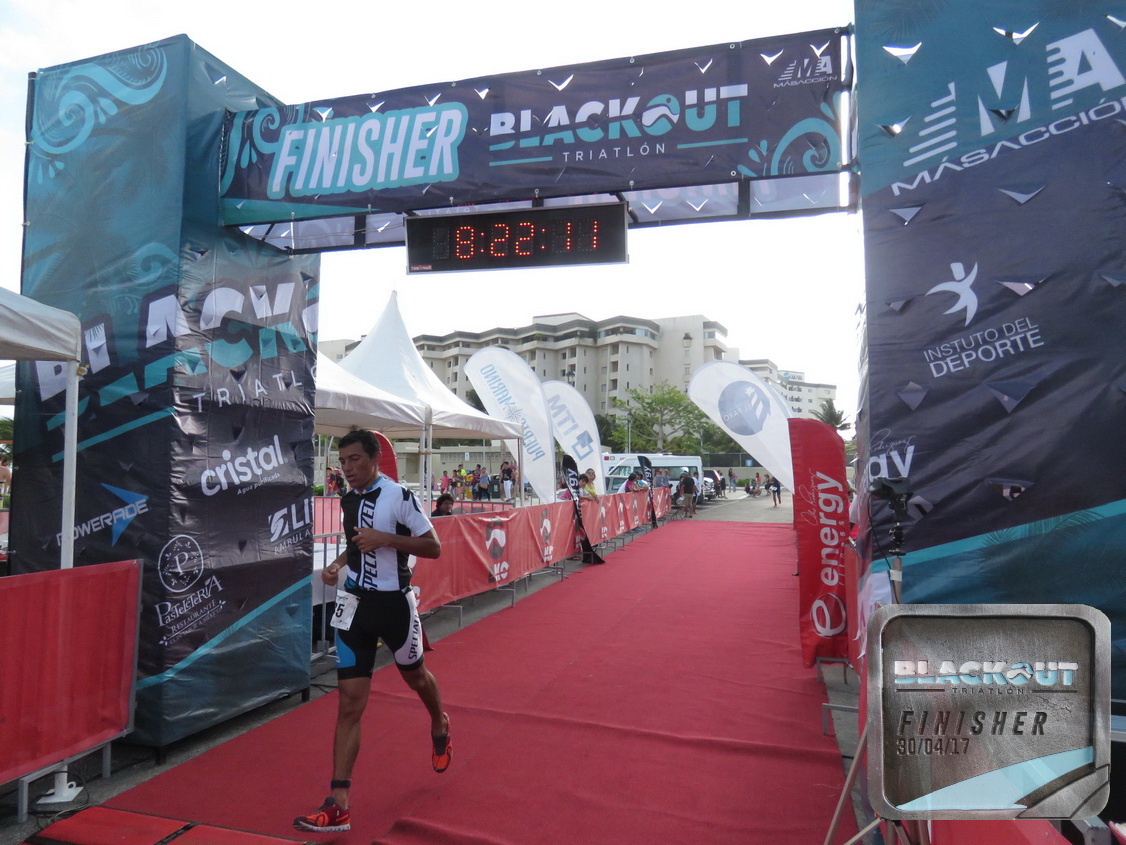The photograph captures the finishing area of a race event, prominently marked by a gateway structure. This structure, with two vertical columns and a connecting horizontal beam, features white text that reads "Finisher" and "Blackout Triathlon." Hanging from the beam is a digital display showing the time "8:22:11." The ground within this gateway area is covered with a red carpet. A male runner, clad in black and white attire with orange running shoes, is seen sprinting on this carpet, having just passed the finish line.

The scene is set outdoors on a bright yet overcast day, under a white sky. Flanking the running area are white tents and multiple banners and posters, indicating the organized nature of the event. On the left side of the image stands a large building, possibly a hotel. Spectators can be seen in the background, standing behind guardrails, immersed in the excitement of the race's conclusion.